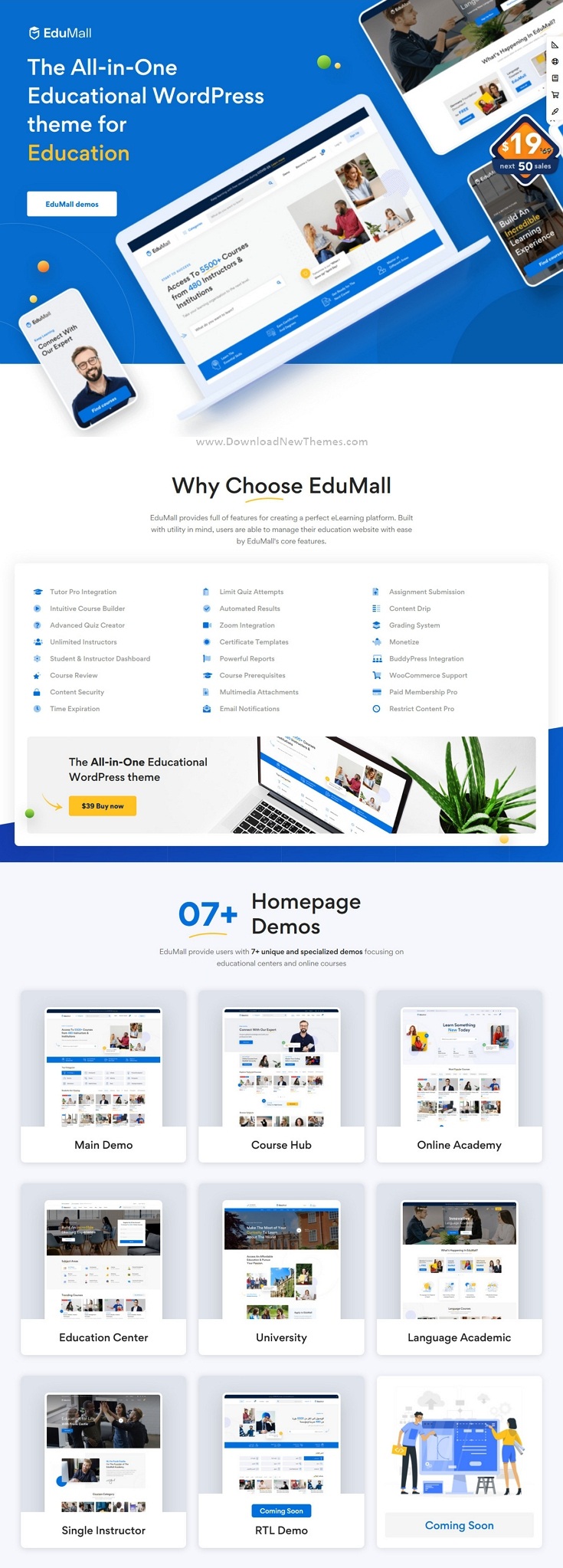Screenshot of EduMall Landing Page

The screenshot captures the vibrant landing page of the EduMall website, designed as an All-in-One Educational WordPress Theme. The layout is visually striking, featuring a diagonal arrangement of various electronic devices, including a cell phone, laptop, and desktop, all in sleek white. This dynamic display contrasts against a bold blue background.

Prominently displayed in white text at the center of the page is the tagline: "The All-in-One Educational WordPress Theme for Education." Just beneath this heading, another line in white reads, "Why Choose EduMall?" accompanied by three sections each marked with blue icons, succinctly outlining the key benefits of the theme.

The lower section of the image showcases a banner with an arrow pointing towards a yellow box, drawing attention to a highlighted feature or call-to-action. Bordering this entire section is a blue outline, above which the text "Homepage Demos 07 Plus" is written in a distinct blue font.

Further down, there is a grid of nine boxes, each presumably showcasing different homepage variations appropriate for various educational institutions, such as education centers and online academies. Due to the screenshot's resolution, the details in these boxes are small and somewhat illegible, but they hint at the diverse range of designs available within the EduMall theme.

Overall, the image illustrates an appealing and functional presentation of EduMall’s educational theme offerings, with a clear and organized layout that highlights its key features and diverse customization options.